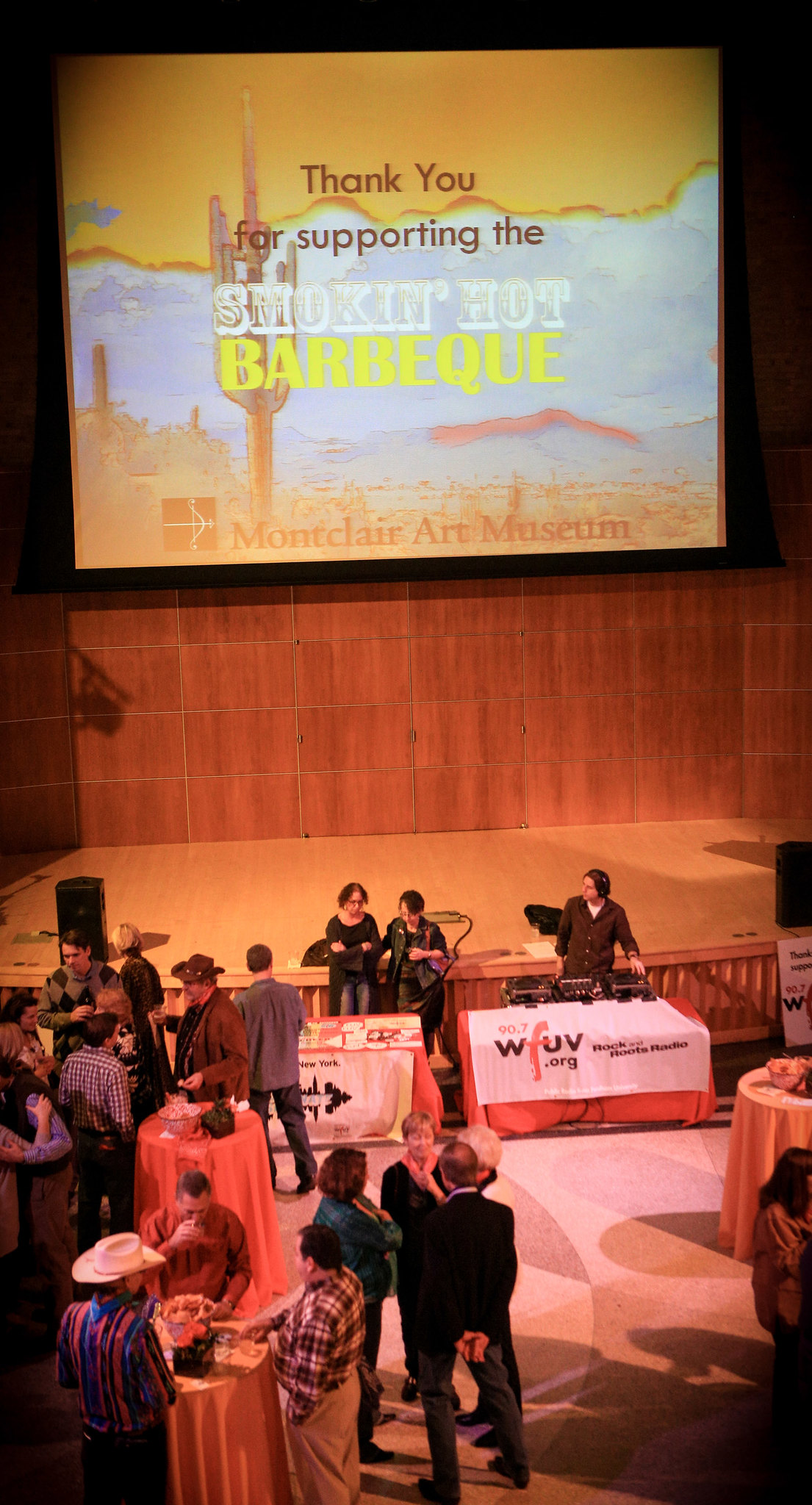The indoor photograph showcases an event set at the Montclair Art Museum, featuring a stage and a projector screen that displays the message, "Thank you for supporting the Smoke and Hot BBQ," with the museum's logo to the left. The stage, adorned with a brown hardwood floor and backdrop, is surrounded by round tables draped in a mix of red and orange tablecloths. The tables are scattered around the area, where people are seen mingling, eating, and drinking. Notable attendees include individuals wearing cowboy hats and a man in a brown jacket, lending a Western theme to the gathering. In front of the stage, there are long rectangular tables covered with banners that read "WFUV.org Rockin' Roots Radio," indicating the presence of presenters, possibly including a DJ with his equipment. The room's decor features a backdrop illustration resembling a desert landscape with cacti and mountains, enhancing the thematic ambiance of the event.